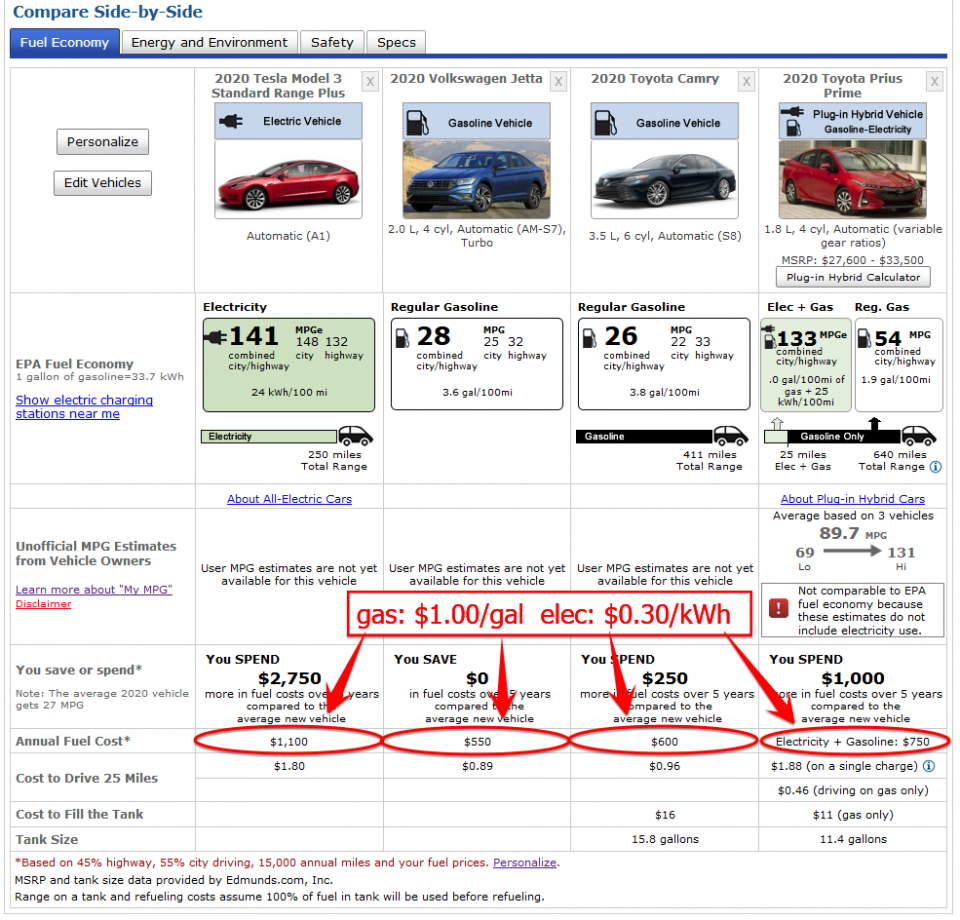In the upper left corner of the image, there's a text label saying "Compare Side by Side." The image is filled with details about various vehicles. Below this title, there are several tabs labeled "Fuel Economy," "Energy and Environment," "Safety," and "Specs." All tabs are gray with black font except for the "Fuel Economy" tab, which is highlighted in blue with white text, indicating the current active section.

The image showcases a comparison of four cars: the 2020 Tesla Model 3 Standard Range Plus, the 2020 Volkswagen Jetta, the 2020 Toyota Camry, and the 2020 Toyota Prius Prime. Each vehicle has detailed listings of their various attributes under the highlighted "Fuel Economy" section.

A box at the bottom of the image lists the costs for gasoline and electricity, highlighted with red font and borders. The costs are indicated as $1 per gallon for gasoline and $0.30 per kilowatt-hour for electricity. An arrow originates from this box, pointing to the annual fuel costs estimated for each vehicle:
- Tesla Model 3: $1,100
- Volkswagen Jetta: $550
- Toyota Camry: $600
- Toyota Prius Prime: $750 (combining electricity and gasoline costs)

Each of these numbers is clearly designated, giving viewers a comprehensive understanding of the annual fuel expenditure for each vehicle included in the comparison.